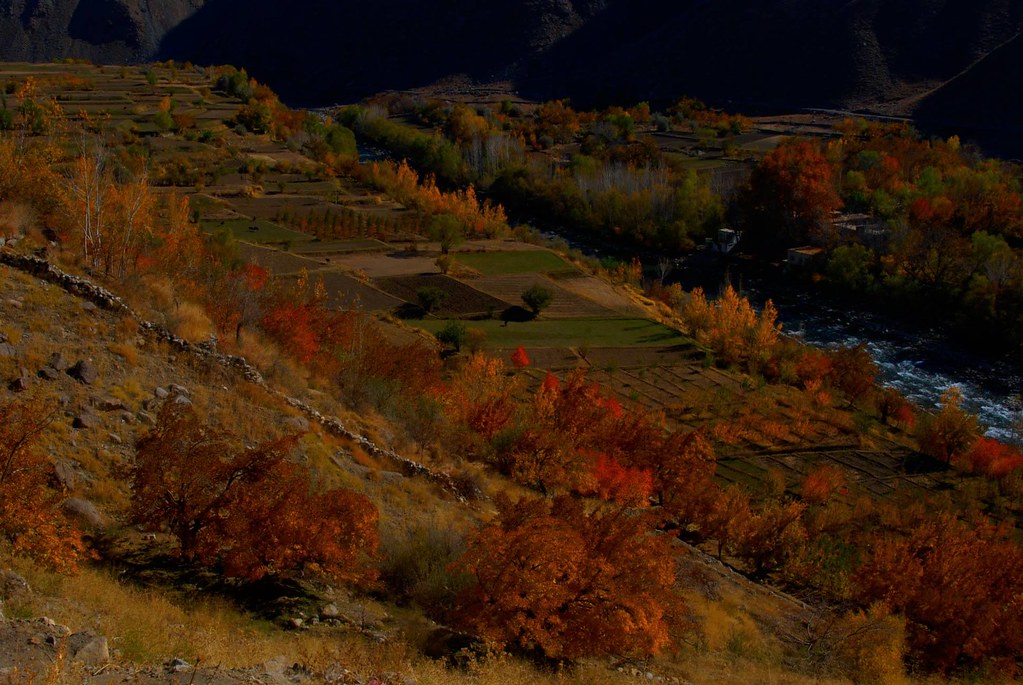The aerial photo captures a sweeping autumnal landscape taken from a helicopter or plane, looking down over a hilly region transitioning into a valley. The foreground on the bottom left corner is rocky with clusters of orange bushes. As the terrain slopes downward towards the center and upper right, an array of vibrant foliage emerges, showcasing a palette of yellow, orange, green, and red bushes interspersed among the fields. Particularly on the left side, there are well-plotted green and brown squares of farmland, meticulously mowed or plowed, with rows of newly planted trees adding to the texture of the vegetation. In the upper right section of the image, a serene stream or lake with blue water meanders through the landscape, further enhancing the contrast of natural colors. Hovering above in the top left, a stark presence of black mountains or perhaps dense shadowed areas forms a dramatic backdrop, underscoring the multifaceted beauty of the countryside in autumn.